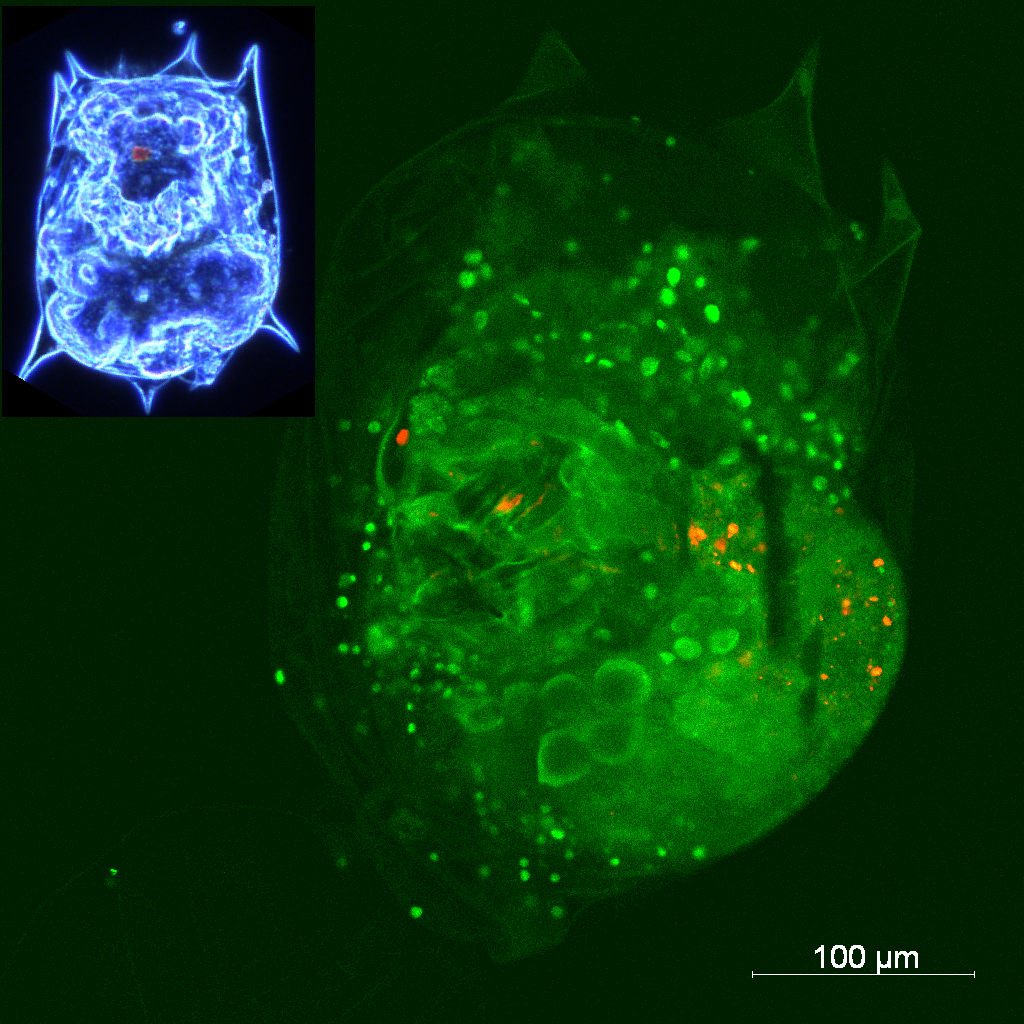This microscope image showcases two translucent, blob-like organisms set against a black background. The primary organism, located in the bottom right, is a green mass with a somewhat gelatinous texture, containing multiple smaller green structures that resemble algae. In contrast, the upper left corner features a similar, smaller organism, but in blue, with hues ranging from light to dark blue and filled with a gloopy, neon substance. Both organisms exhibit features that might remind one of ghostly or jellyfish-like entities, with the green one notably bearing a resemblance to Slimer from Ghostbusters. The image includes a scale marker indicating 100 nanometers, providing a sense of the organisms' microscopic size, and occupies a relatively small portion of the frame.